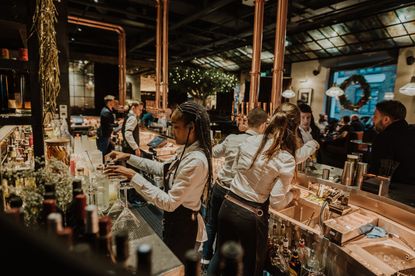This image captures the bustling interior of an upscale bar during the Christmas season. At the center of the scene, five bartenders—three women and two men—are meticulously mixing drinks and attending to patrons. All the bartenders are dressed in white shirts, black aprons, and black bottoms, presenting a coordinated and professional appearance. The two women on the left side of the bar have their hair pulled back, while one has long braided hair. They are engaged in various tasks such as mixing drinks and possibly writing orders. The counter spans both the front and back of the bartenders, adorned with bottles and other bar essentials. 

In the background, the bar area is tastefully decorated with a large Christmas wreath hanging against a window, which brings in some natural light from overhead windows. Additionally, long copper pipes hanging from the ceiling add to the bar's aesthetic appeal. Light fixtures are scattered throughout the space, enhancing the cozy yet vibrant atmosphere. Various patrons are seated and mingling at the bar, reinforcing the lively environment.